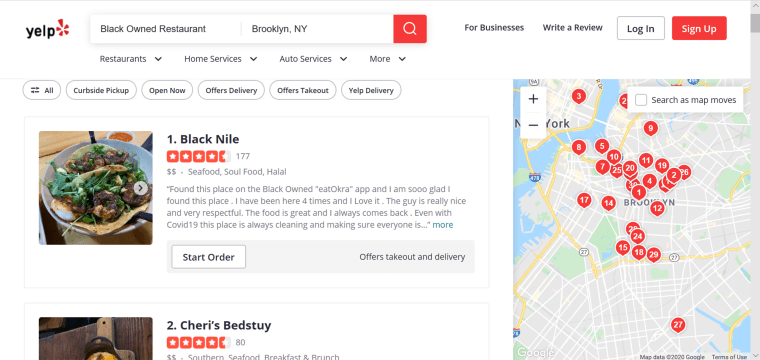The image displays a Yelp page showcasing restaurant listings. On the right side of the page, there is a map highlighting various locations in New York City, each marked with small red balloons containing numbers. The top left corner of the map includes an option labeled "Search as map moves."

Two restaurant listings are prominently shown: Black Nile and Sherry's Bed-Stuy. Black Nile has a detailed review which reads: "Black Nile - 4.5 stars. Specializing in seafood, soul food, and halal dishes. Discovered this place on the Black-owned Eat Okra app and I am thrilled I did. I've visited four times and absolutely love it. The owner is incredibly nice and respectful, the food is fantastic, and I always return. Even during COVID-19, this restaurant maintains strict cleanliness protocols, ensuring the safety of all patrons." An option to read more of the review is available.

The image effectively illustrates the user interface of Yelp, complete with interactive map features and detailed customer reviews.